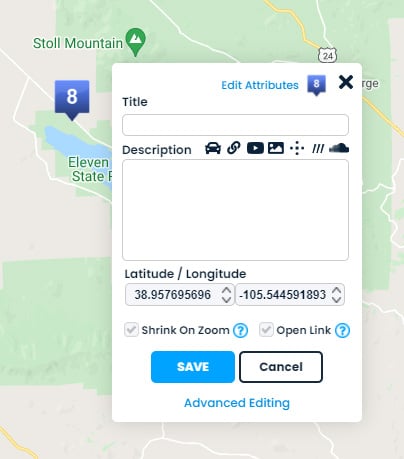The image is a screenshot from a Maps app featuring Stoll Mountain. In the upper left, a map is visible with "Stoll Mountain" labeled in green, surrounded by a white border. The map includes a pin icon indicating a mountain location. Beneath this, a blue number eight with a pointed end is partially visible. Below this, a green label reads "11 state," though part of the text is cut off. 

Overlapping this is a white rectangle labeled "Edit Attributes" in light blue at the top right. Adjacent to this label is a blue shape with another pointed-eight symbol, followed by a bold, black "X." Below this, fields for "Title" and "Description" are visible. 

The "Description" section includes icons representing a car, a link, the YouTube logo, an image, a cross-like intersection, three dashes, and a cloud, with space to write a description of the trip. Below, "Latitude - Longitude" is written in dark gray with two dropdown menus displaying "38.957695696" and " -105.544591893," respectively.

Additional options include a light gray checked box labeled "Shrink on Zoom" with a blue question mark inside a blue circle next to it. Another light gray checked box is labeled "Open Link," accompanied by a blue check mark inside a blue circle. At the bottom of the white rectangle are two buttons: a blue, rounded rectangle labeled "Save" in white lettering and a "Cancel" button with a black border.